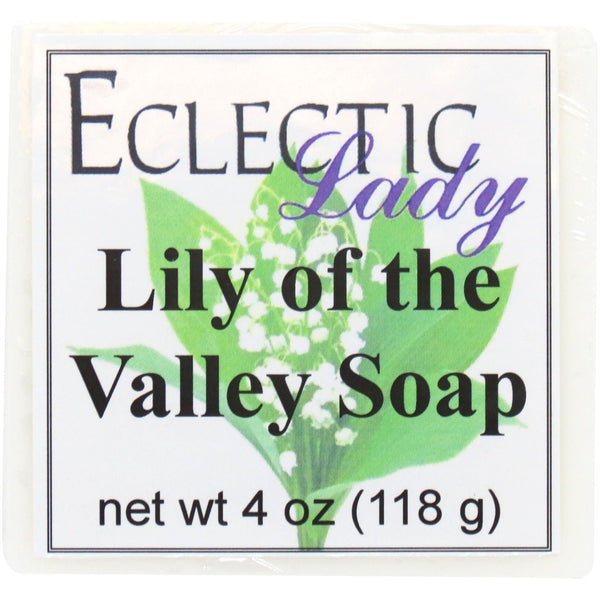The image features a label for Eclectic Lady Lily of the Valley Soap, with a net weight of 4 ounces (118 grams). The label itself is set against a white background, adorned with an image of a lily of the valley flower. The text "ECLECTIC" is printed in all caps using a black font, while "Lady" appears in a cursive, lavender or purple font. "Lily of the Valley" is written in a plain New Times Roman font. The entire label is outlined by two thin black lines forming a square frame. The design includes a green leaf with white flowers at the center, adding to the natural aesthetic. The simplistic yet elegant design suggests it may be an advertisement or a visual representation typically found on the soap's packaging.